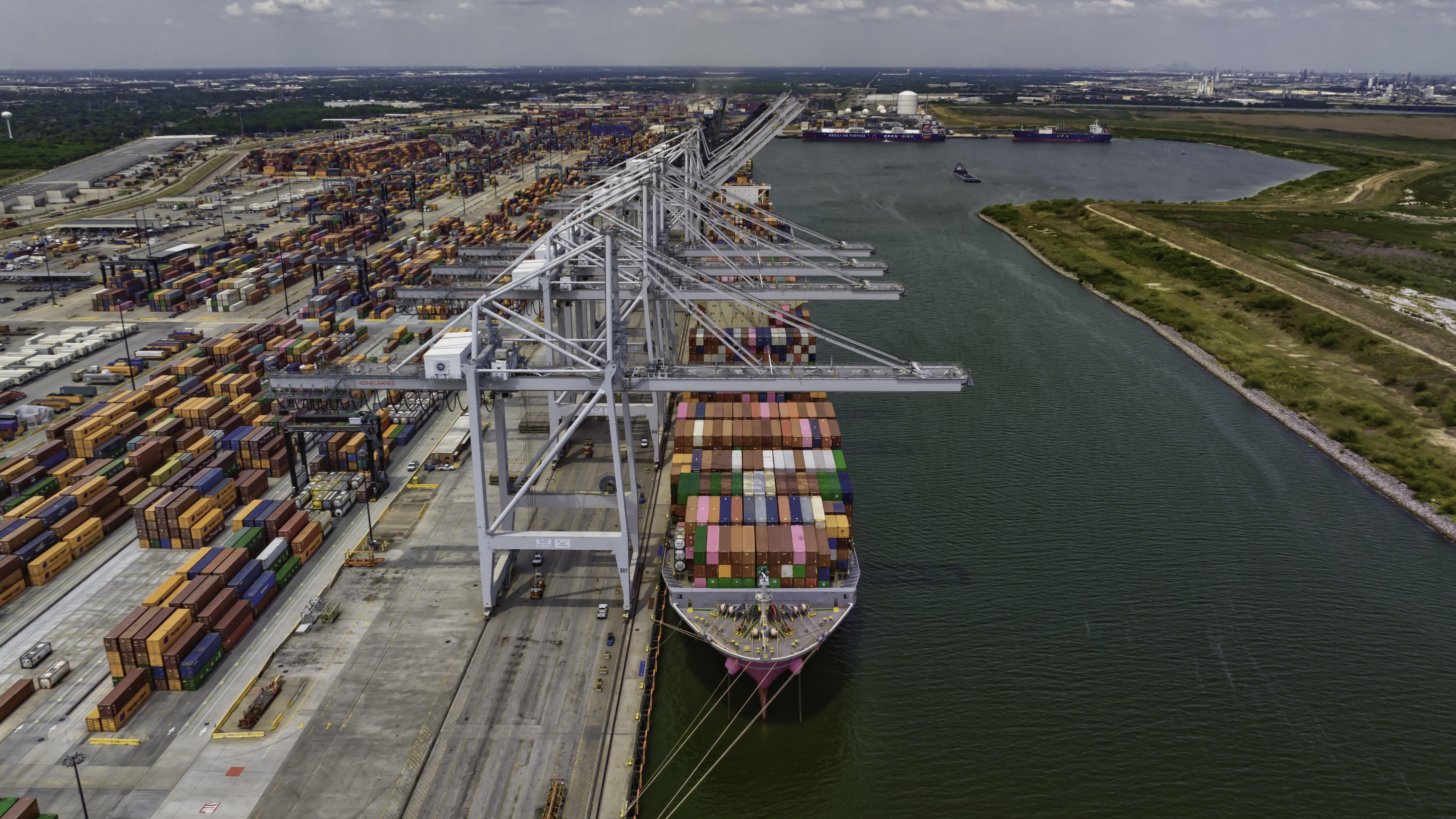The daytime aerial photograph captures a bustling shipping dock with vibrant blue skies and minimal clouds. Dominating the foreground is a large ship stacked with multi-colored shipping containers in hues of blue, rust, yellow, and green, docked at a port. The left side of the image features a multitude of containers being loaded and unloaded by prominent cranes, adding an industrial flair to the scene. On the right-hand side, the landscape transitions to lush greenery and grass, followed by a broad waterway or canal. In the distance, a few more ships patiently await their turn at the dock. 

In the background, a city skyline emerges faintly amidst some green fields and trees, contributing to the image's intricate blend of natural and urban elements. The right side of the image includes a panorama of expansive waters, enhancing the scene's depth and emphasizing the port's strategic location. Overall, this descriptive snapshot intricately frames the dynamic operations of a cargo handling zone within a serene, yet industrious landscape.